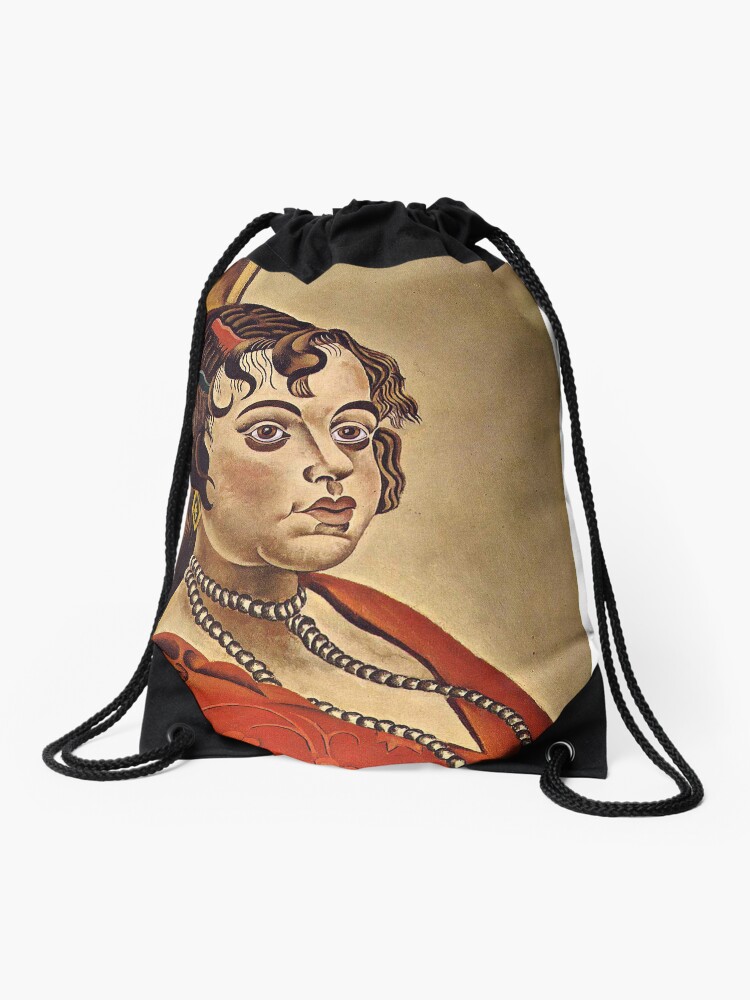This image depicts a black drawstring bag, centrally placed against a white background. The bag features a detailed portrait of a woman in a style reminiscent of classical or medieval painting. The woman, facing slightly to the left, has a rounded face with curled, coiffed brown hair tinged with red. She is adorned with a double-looped necklace of white pearls and dons a low-cut red blouse that reveals her neckline. The dominant colors in the image include black, red, brown, white, gray, and beige. There is no text visible on the bag, and the overall composition highlights the intricate design on the bag which creates a rich visual focus.